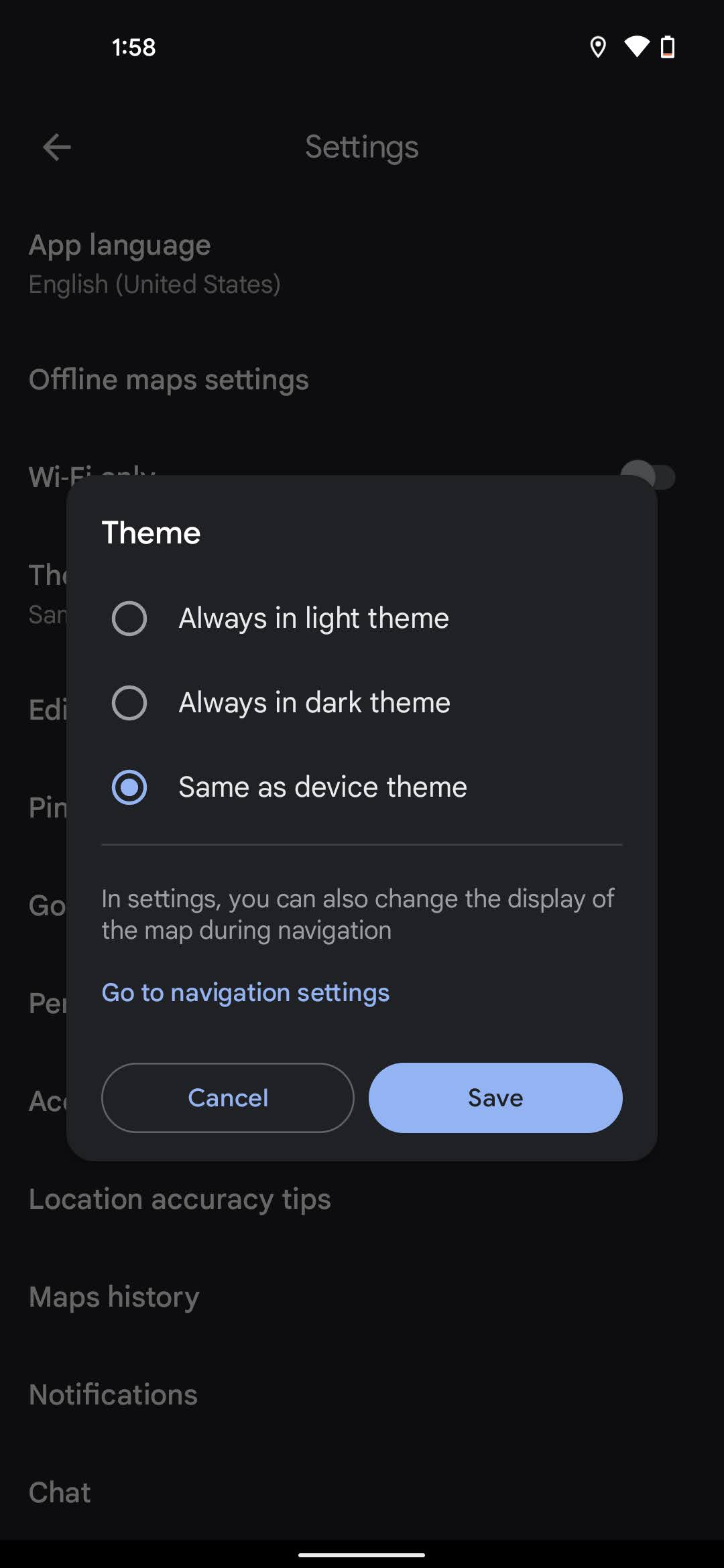Screenshot of an Android phone settings interface displayed in dark mode. The "Theme" option within the settings shows three choices: "Always in light mode," "Always in dark mode," and "Same as device theme," with the latter currently selected. The text indicates that users can change the theme for map display during navigation by going to the navigation settings. The options to "Cancel" and "Save" are highlighted in blue. In the background, various other Android settings are visible, contributing to the overall dark mode aesthetic.